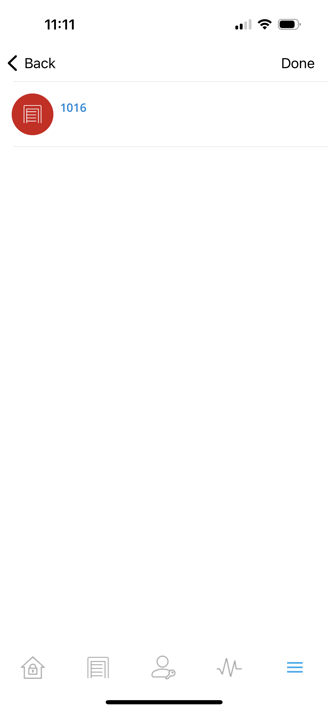This image is a screenshot of an application on a mobile device, likely an iPhone, given the visible status and notification bars at the top. It is 11:11, though it's unclear whether it's AM or PM. The device shows a mid-level cellular reception with two bars, full Wi-Fi reception, and approximately 80% battery life.

The background of the app is predominantly white, blending seamlessly with the surrounding margins of the image. At the top of the screen, there is a navigation bar. On the left side of this bar, there is a "Back" button accompanied by a left-pointing arrow, while on the right side, there is a "Done" button.

Below this bar, the primary content of the screenshot features a single red circular icon with a document logo. This icon is aligned with the text "1016." The rest of the screen is blank, making up about 70% of the visual space.

At the bottom of the screenshot, there is a navigation menu with several icons: a home icon, a document icon, an icon resembling a person's head, an icon that looks like an EKG meter, and finally, a menu bar icon. This detailed layout suggests that the app might be some kind of organizational or productivity tool.